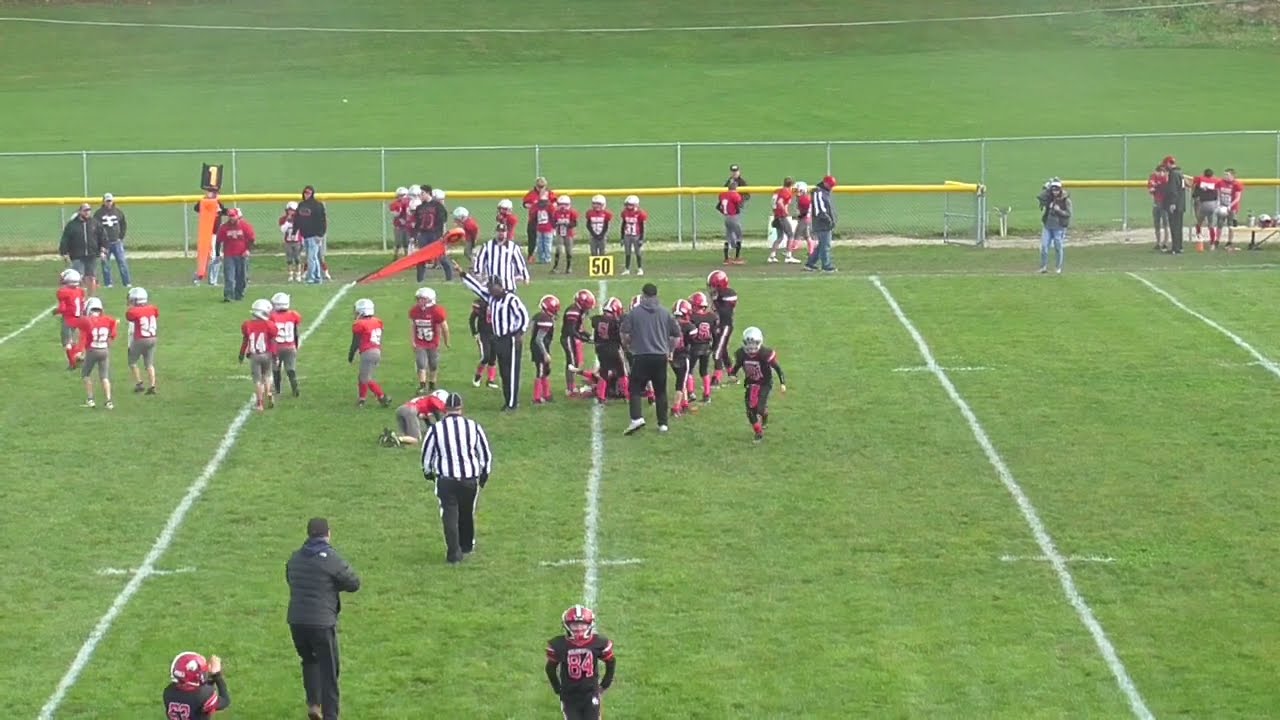The image captures a youth football game in progress on a vibrant green grass field marked with white yard lines. The scene is set at the 50-yard line, where most of the action is taking place. One team is dressed in red jerseys, white helmets, and gray pants, while the opposing team sports black jerseys, black pants, and red helmets. Three referees in traditional black pants and white-striped shirts are seen on the field, with one signaling a first down. Coaches and a few adults stand by, engaging in their roles, with kids either on the sidelines or actively involved in the play. A yellow-topped soft padding fence runs along the perimeter, beyond which is a taller fence enclosing more green space and possibly another fence further in the background. The scene underscores the community atmosphere with players, referees, coaches, and a sparse presence of parents or spectators, demonstrating the dynamic yet organized nature of the game.